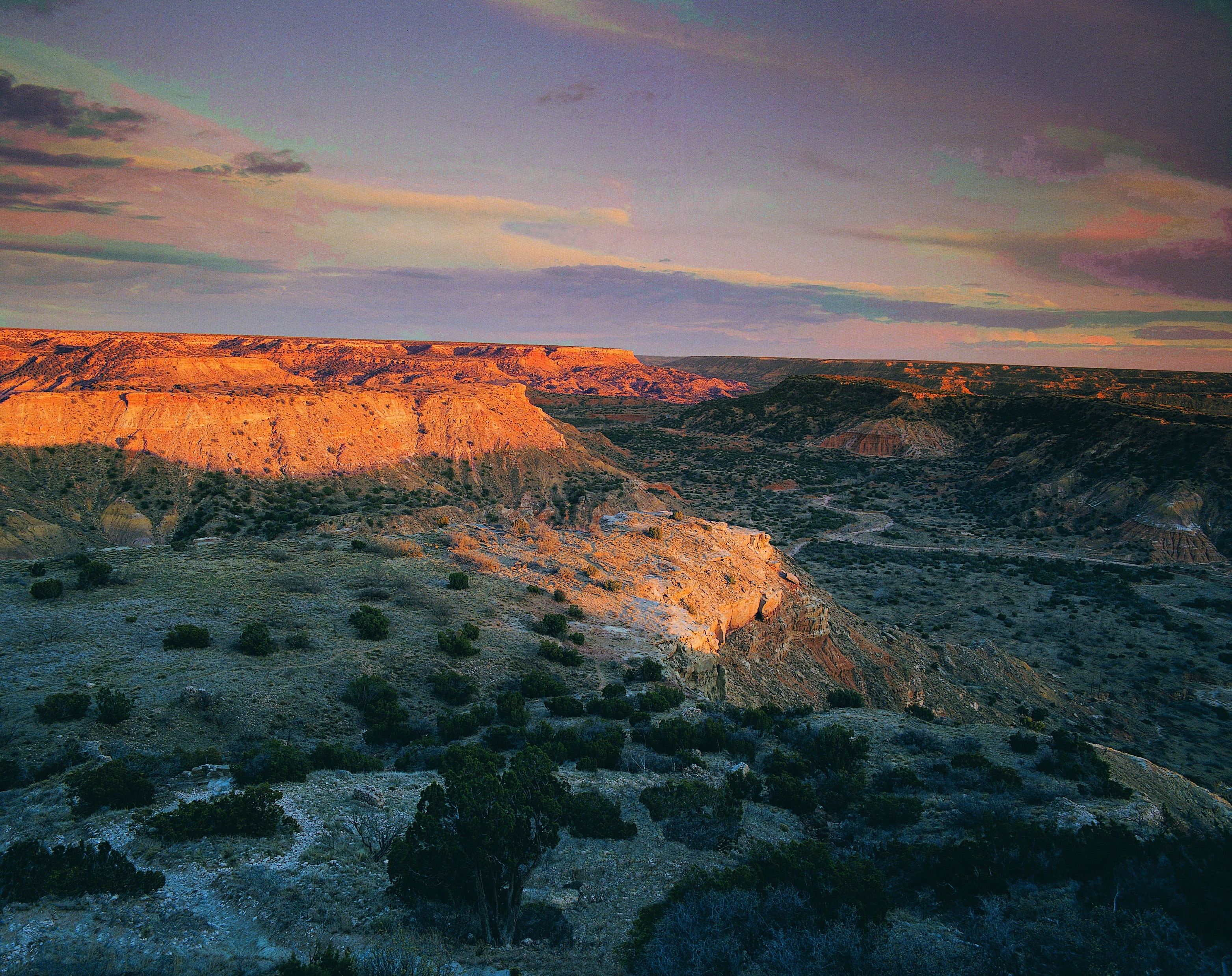This image captures a breathtaking sunrise or sunset over a canyon, likely the Grand Canyon or a similar geological region. The sky is a mesmerizing blend of colors, transitioning from vibrant oranges and purples to subtle greens and grays, with light clouds stretched like cotton candy across the horizon. The photograph, seemingly taken from a high vantage point, possibly by a drone, showcases the canyon's rugged landscape, illuminated beautifully by the sun's light. The orange-tinted canyon walls are prominent in the upper left portion of the image, with shadows casting a dramatic contrast across the valley. A dried riverbed cuts through the scene from the lower right to the center top, adding a dynamic element to the composition. Sparse vegetation, including small bushes approximately 10 to 15 feet apart, dots the landscape, and flat-topped mountains or ridges dominate the view. In the middle of the image, a road or trail meanders through the valley, hinting at human interaction with this otherwise wild and expansive desert terrain.